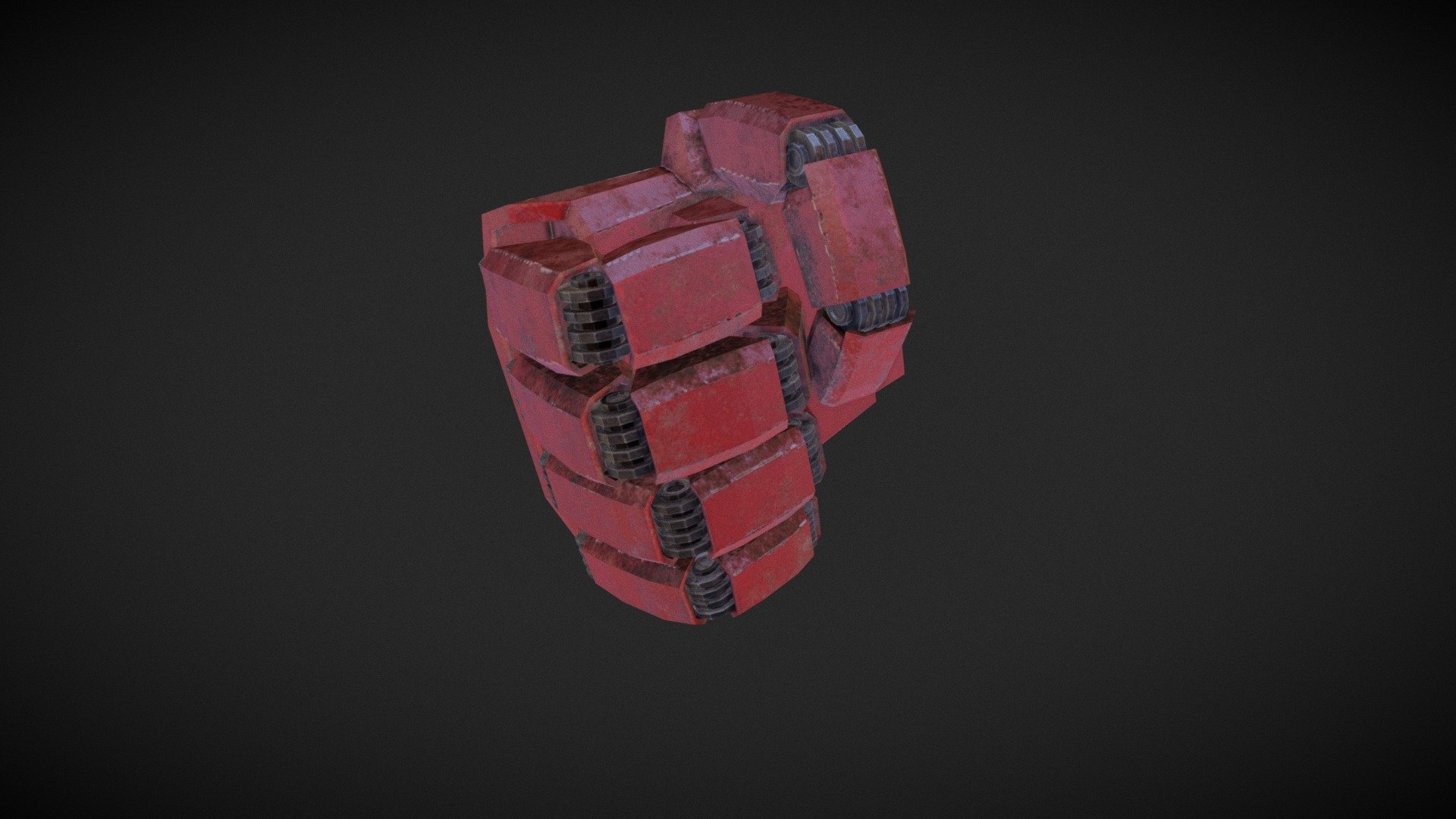The image features two weathered red metal objects on a solid black backdrop. The primary object, prominently displayed and slightly angled to the right, is a thicker structure composed of four separate red compartments. Each compartment has four black hinge-like features positioned in a spaced-out manner, giving the impression of integrated mechanisms. The second object, partially obscured behind the first, is thinner and oriented sideways, showing only about a quarter of its structure. Similar to the first object, it has four black clasp-like devices along its edges. Both objects exhibit a distressed appearance, suggesting they are well-used components, possibly parts of a machine or motor. The detailed and cohesive arrangement of hinges and clasps indicates they likely function together, possibly engaging with gears or similar mechanisms.